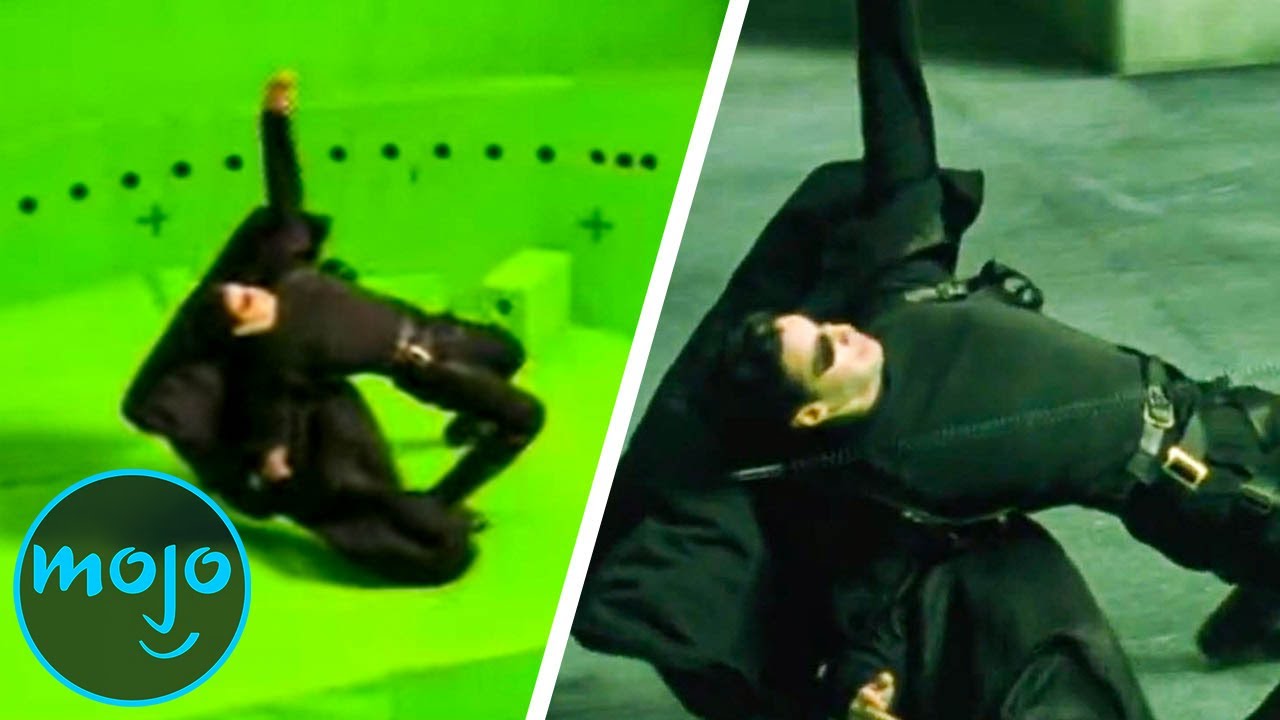This image contrasts two different views of a famous scene from The Matrix where Neo, played by Keanu Reeves, is dodging bullets in slow motion. On the left side, we see the actor Keanu Reeves in a green screen setup, his knees bent and one arm stretched out with a black cape flying behind him. The background is bright green with black dots, indicating a special effects area. In the bottom left corner, a circular logo with 'Mojo' in blue text is visible, suggesting this image is a screenshot from a YouTube video by the Mojo channel. On the right side, a closer shot from the film shows Neo's intense concentration as he leans back to dodge a bullet, sunglasses on, all dressed in black. This background appears more natural, resembling stone or concrete, highlighting the shift from the green screen creation to the final movie scene.